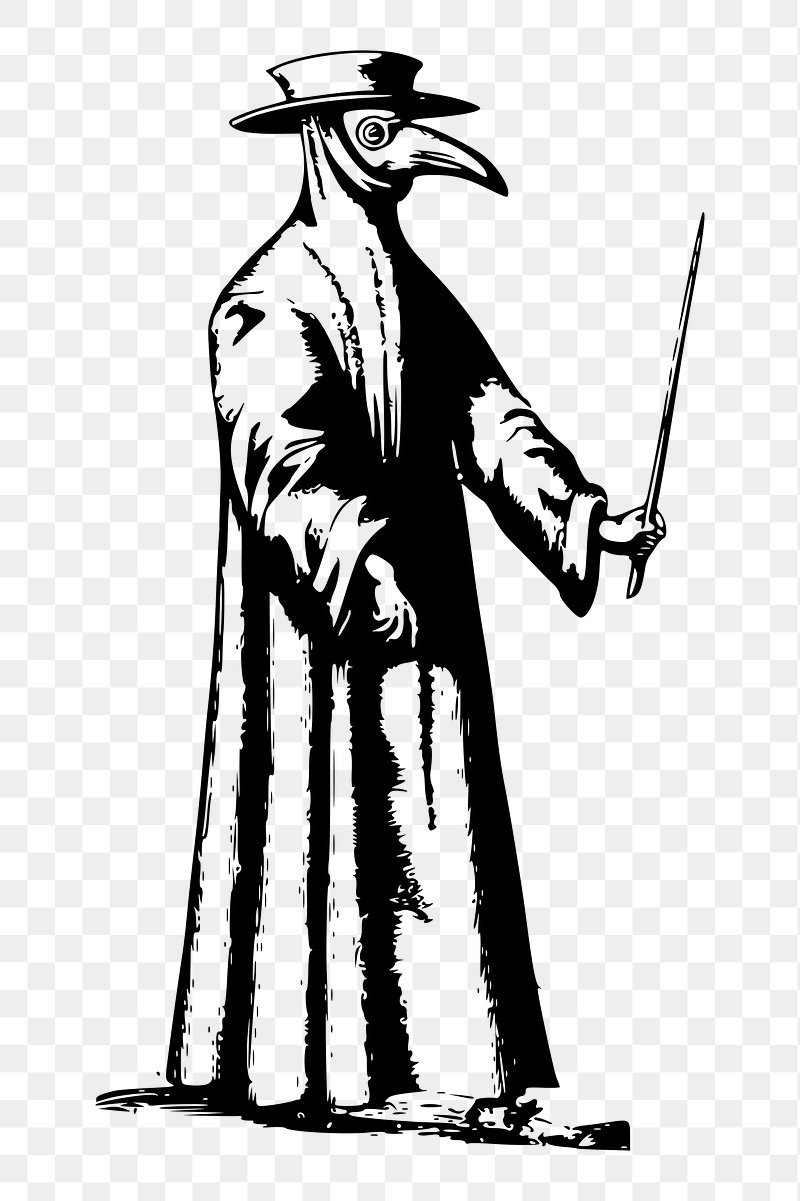In this image, there is a detailed, black and white sketch of a character with a bird-like head, complete with a long beak and an eye visible beneath a top hat adorned with a larger rim. The character is captured in a mid-walk, side view, dressed in a full-length robe that extends down to the feet and also wraps around most of the face. Human hands emerge from the robe; the left hand holds a stick, baton, or pointer raised towards the sky, while the right hand is empty. The background features a repeating checkered pattern of light blue and white squares, adding a subtle contrast to the monochrome drawing.